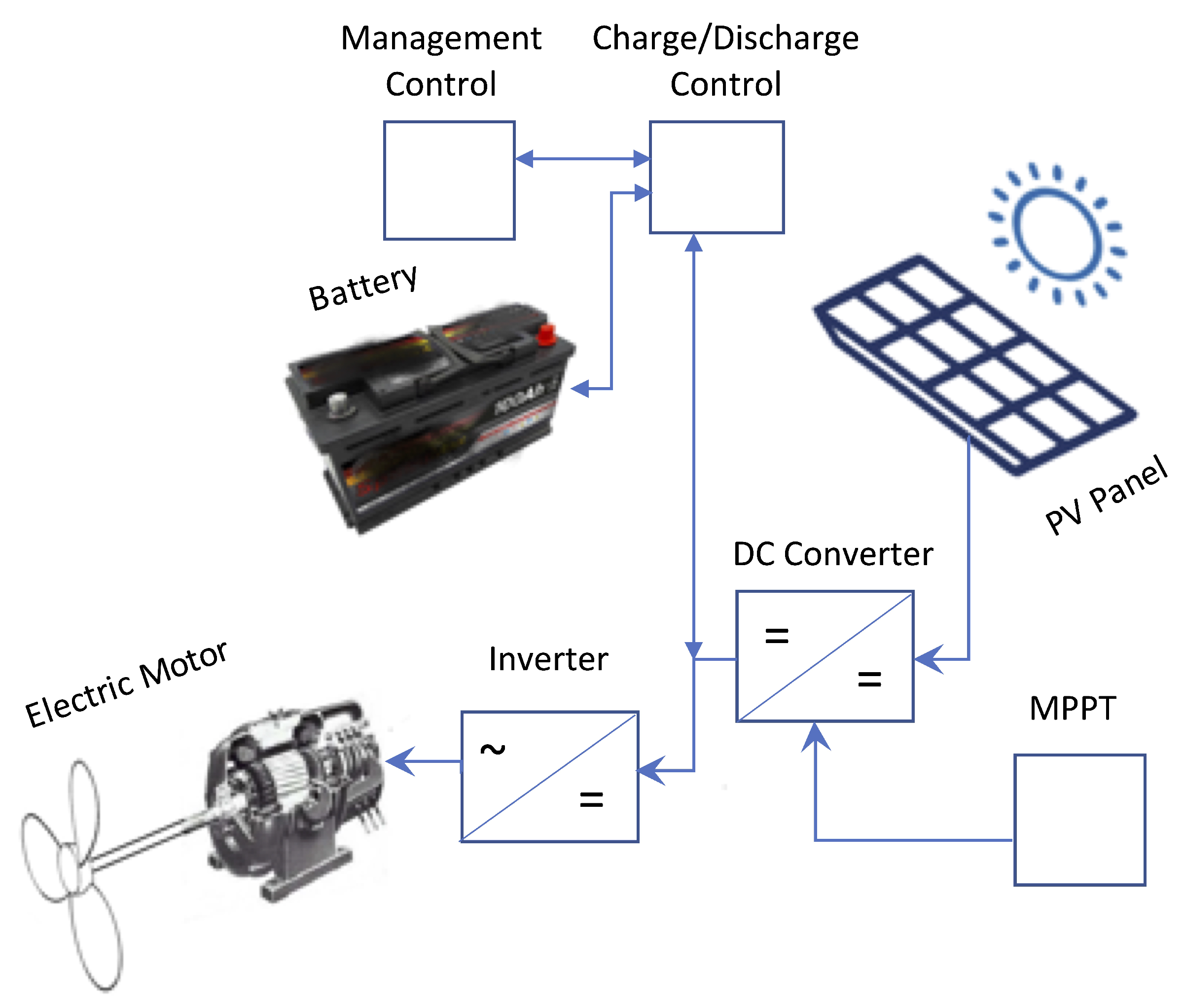This detailed technical diagram, primarily in black and white with striking blue elements such as boxes and arrows, provides an instructional overview of an electric motor and PV (photovoltaic) panel system. At the top right, a blue-outline sun adjacent to a grid labeled "PV Panel" depicts the solar power source. Various blue squares and rectangles represent key components, including MPPT (Maximum Power Point Tracking), DC converter, charge/discharge control, management control, battery, and inverter, all interconnected by arrows. Text annotations clarify the function of each part. At the bottom left, an electric motor equipped with a fan blade is depicted, illustrating the flow from solar energy to battery storage and ultimately powering the motor. This flowchart-style diagram emphasizes the order of operations and compatibility within the system, making it ideal for users dealing with battery-powered or solar-powered devices.